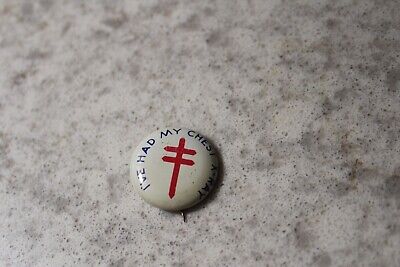The photograph features a small, vintage pin placed slightly to the left and lower than the center of the frame, on a flat surface with a white and gray speckled, marble-like texture. The white pin has blue text wrapping around its circular edge, stating, "I've had my chest x-ray." In the center of the pin is a bold red symbol, resembling a modified equal sign with two horizontal lines intersected by a vertical line. The glossy pin slightly reflects the light, adding a subtle sheen to the image.